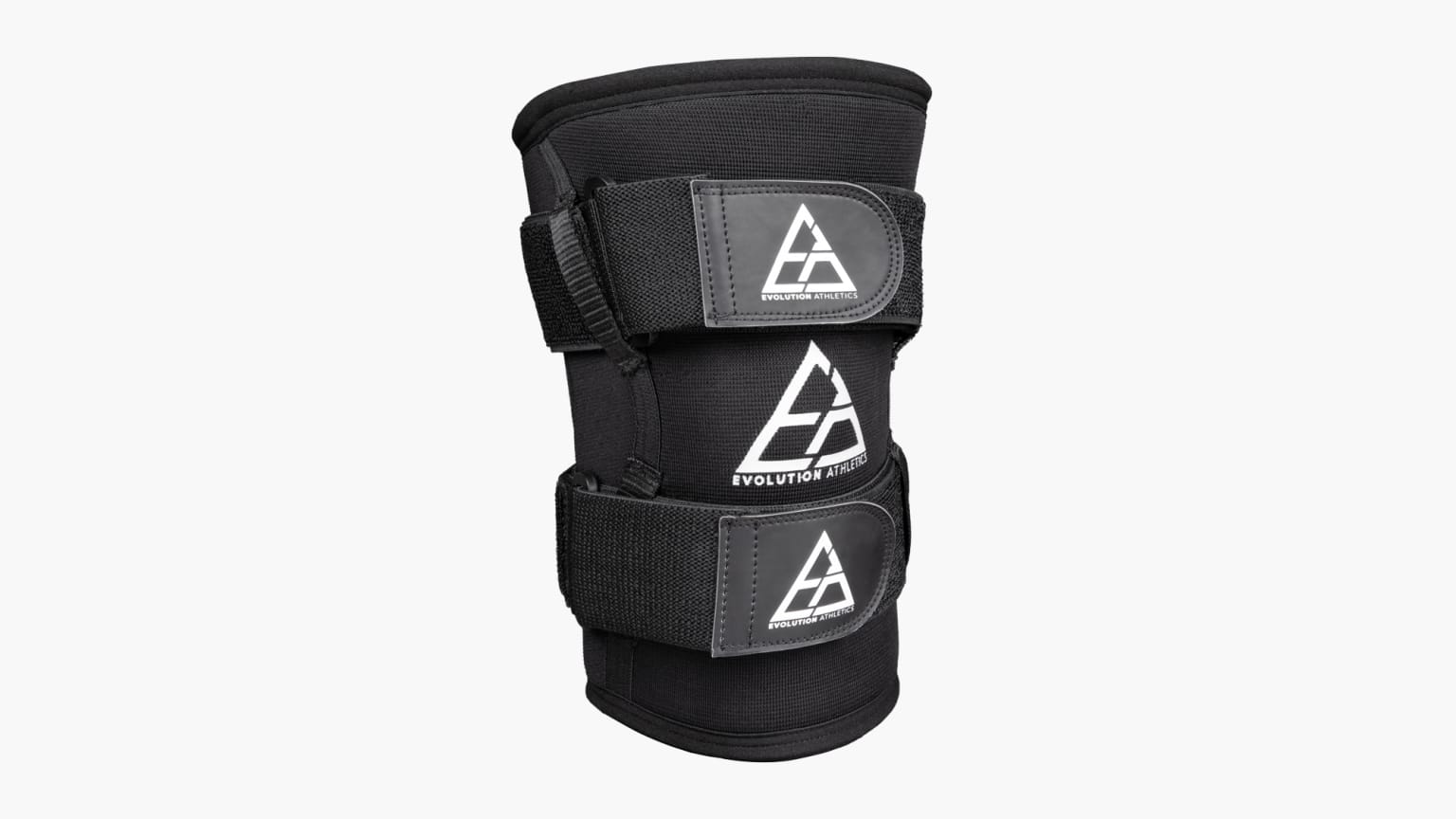The image showcases a black brace, potentially designed for use on either an elbow, knee, or leg, situated against a plain white background. The brace, which tapers slightly in the middle before narrowing towards the bottom, appears to be primarily made of a soft, flexible fabric material. It features two Velcro straps, which may incorporate elements of leather or vinyl, but the Velcro itself isn't visible. Adorning the brace are three white triangular logos with lines running through them, positioned with one logo on each strap and another on the main body of the brace. Beneath each logo, text reads "Evolution Athletics," signifying its brand.